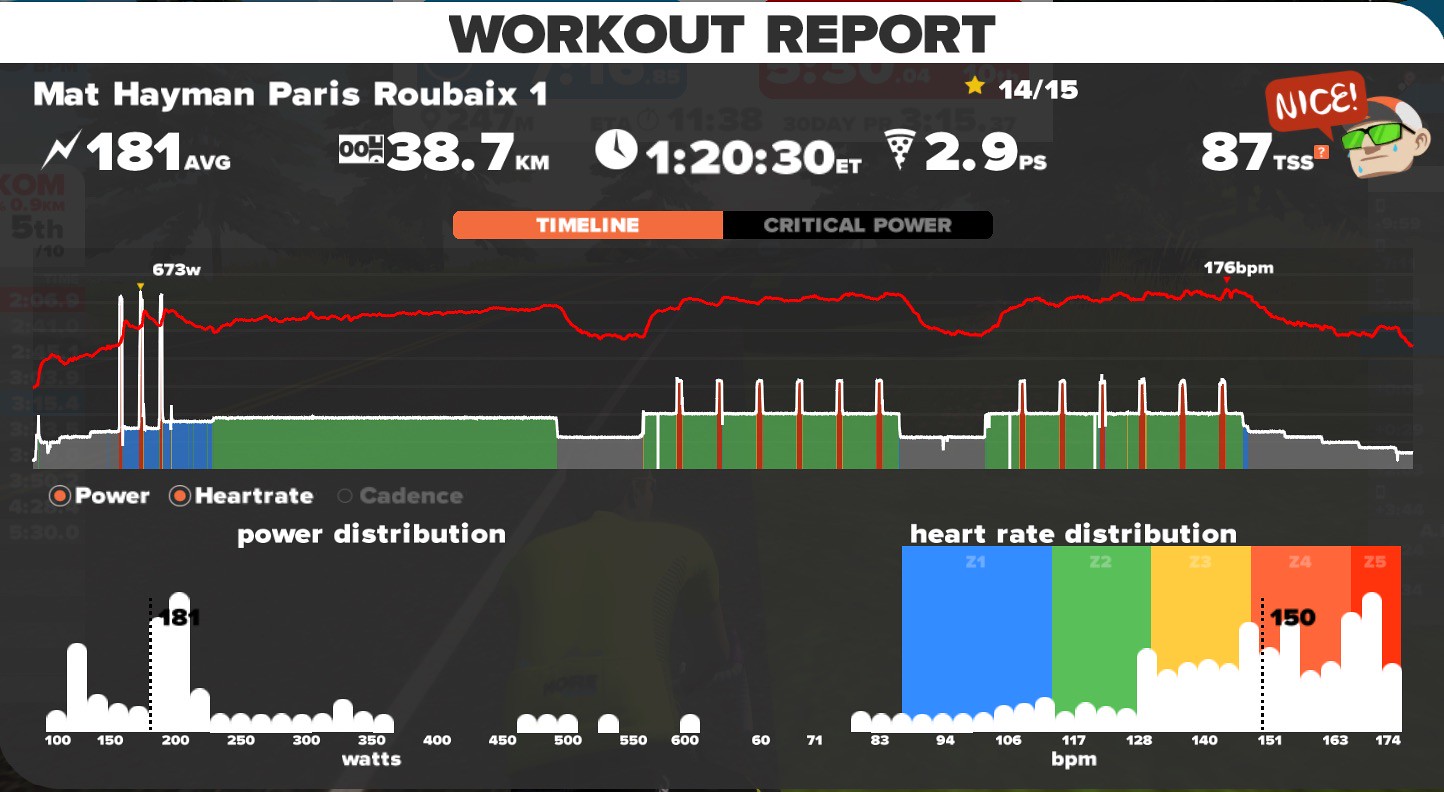The image is a detailed graphic readout from an exercise program or fitness device, possibly on a treadmill. At the top, against a white background with black text, it prominently displays "Workout Report." The central grayish background area features a summary of workout statistics for Matt Heyman during the Paris Roubaix, including "Roubaix number one," "14 out of 15," an average of "181 watts," a distance of "38.7 kilometers," a time of "1 hour, 20 minutes, and 30 seconds ET," "2.9 PS," and a "87 TSS." To the top right, an icon of a man wearing a baseball cap in a red speech bubble says "Nice." Below this, graphical data is illustrated, showing a power distribution graph with values ranging from 637 watts to 176 BPM. Heart rate distribution, displayed on a horizontal bar graph, depicts power, heart rate, and cadence with a jagged red tracking line across sections of blue, green, and gray peaks. The bottom left corner details a power distribution meter, while the bottom right corner highlights a heart rate distribution meter with progress bars in varying colors (blue, green, yellow, orange, red) against a white background. The overall style is a combination of color illustration and graphic design typography in a landscape orientation.